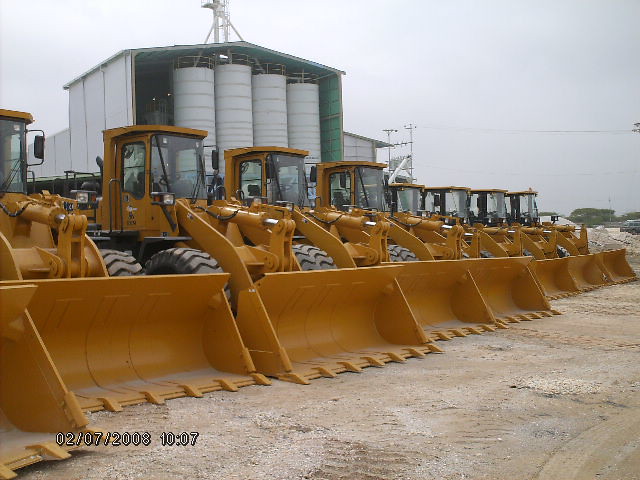This is a detailed photograph taken outside on February 7, 2008, at 10:07 AM, showcasing a lineup of eight large orange tractors equipped with prominent scoops or shovels at their front. The tractors, also described as bulldozers or earthmovers, have massive tires with deep treads and are positioned side by side in a nearly vertical row from the bottom left toward the right of the image. They are set on a pavement with sandy dirt visible at the front. 

In the background, there is a large industrial building with big silos, likely for grain, situated within an enclosure, topped with metal machinery. Electrical lines are running along the side of this structure. A white shed-like building with at least four cylindrical silos inside can also be seen to the left. Additionally, there is a car and a large sandpile visible to the right of the tractors. The sky in the background appears almost white, giving a clear, bright context to the scene.